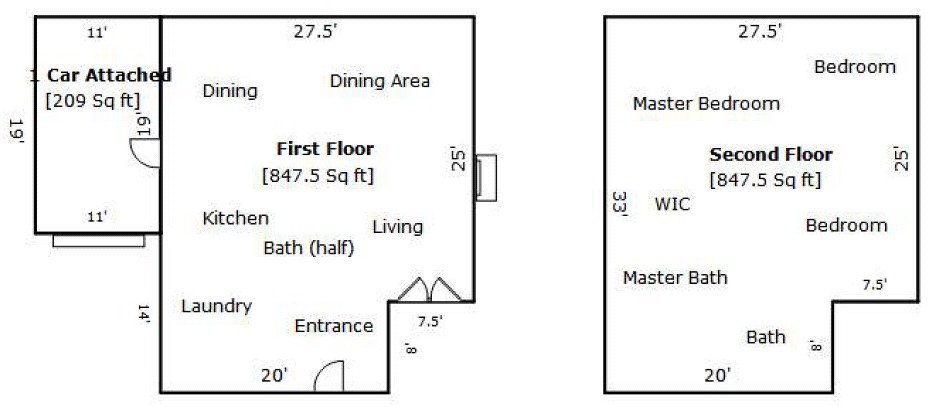This image displays a detailed floor plan of a two-story house, with an adjacent garage area. 

**Garage Area:** 
- Size: 209 square feet, measuring 19 feet in length by 11 feet in width.
- Features: Includes a doorway connecting directly to the first floor.

**First Floor:**
- Total Area: 847.5 square feet.
- Dimensions: The main section spans 27.5 feet in width and 25 feet in depth.
- Features: A small recessed area of 7.5 by 8 feet is situated at the bottom right corner, featuring a double door.
- Rooms: 
  - Dining Area
  - Kitchen
  - Living Room
  - Half Bath
  - Laundry Room
  - Entrance

**Second Floor:**
- Total Area: 847.5 square feet.
- Dimensions: Identical to the first floor with the main area measuring 27.5 feet by 25 feet, including a similar 7.5 by 8 feet recess in the bottom right-hand corner.
- Rooms:
  - Master Bathroom
  - Master Bedroom
  - Bedroom
  - Additional Bedroom
  - Walk-In Closet (WIC)

**Overall Structure:**
- The long edge of the rectangular outline of the plan measures 33 feet.

The well-organized floor plan provides a clear and comprehensive layout of both levels of the house, along with the attached garage.